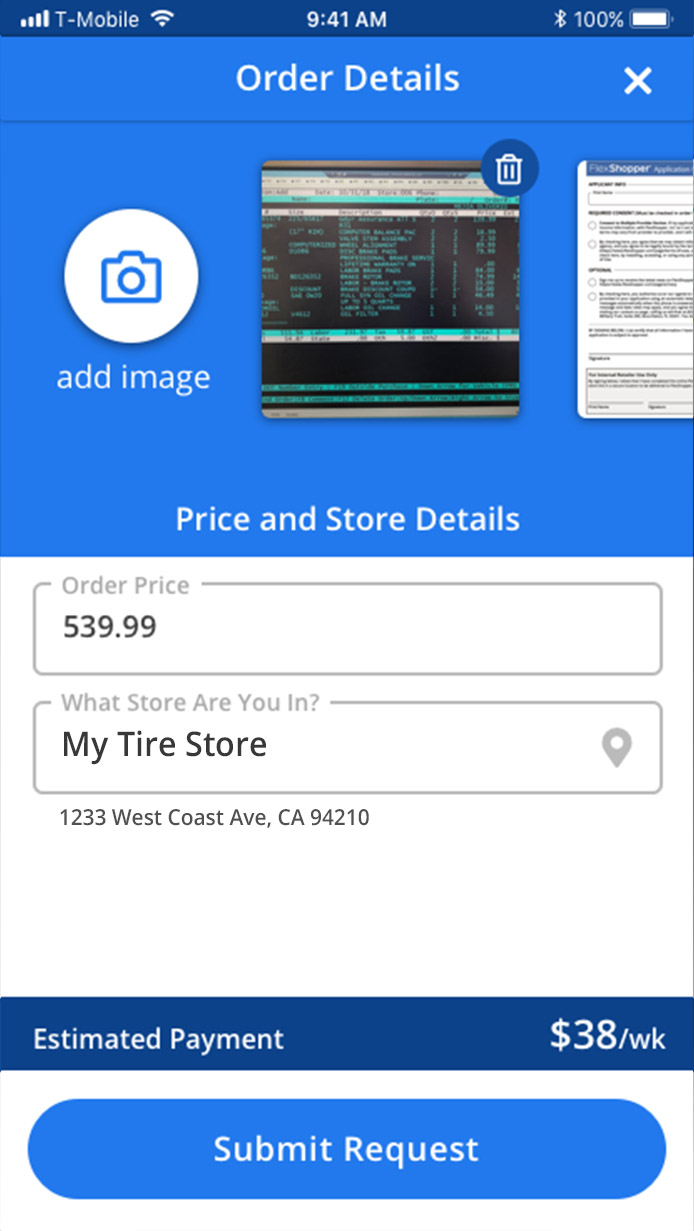In the image, the face of a T-Mobile cell phone is displayed, showing order details for a tire store. The dark blue sliver at the top indicates the T-Mobile network, along with signal bars, Wi-Fi connection status, the time (9:41 AM), and a fully charged battery icon (100% battery life). 

Nearly half of the screen at the top is occupied by a royal blue section providing order details in white font, with a white 'X' in the corner to close this section. There is an option to add an image, although its purpose is unclear. 

Central to the screen is a white document resembling a computer screen icon displaying order details, including a garbage can icon presumably for deletion. Below this, the text "price and store details" is in white font.

In the middle third of the screen, a white background features several gray outlined boxes. Prominently, in black text, the order price of $539.99 is shown. Beneath the text "What store are you in?" is the store name, "My tire store," accompanied by a directions icon for mapping the location. Further down, the store address is listed as "1233 West Coast Avenue, California, 94210."

Near the bottom of the screen, a navy-blue box displays an estimated payment plan of $38 per week. Finally, a large, oblong, rounded royal blue button labeled "Submit Request" can be clicked to finalize the tire order request.